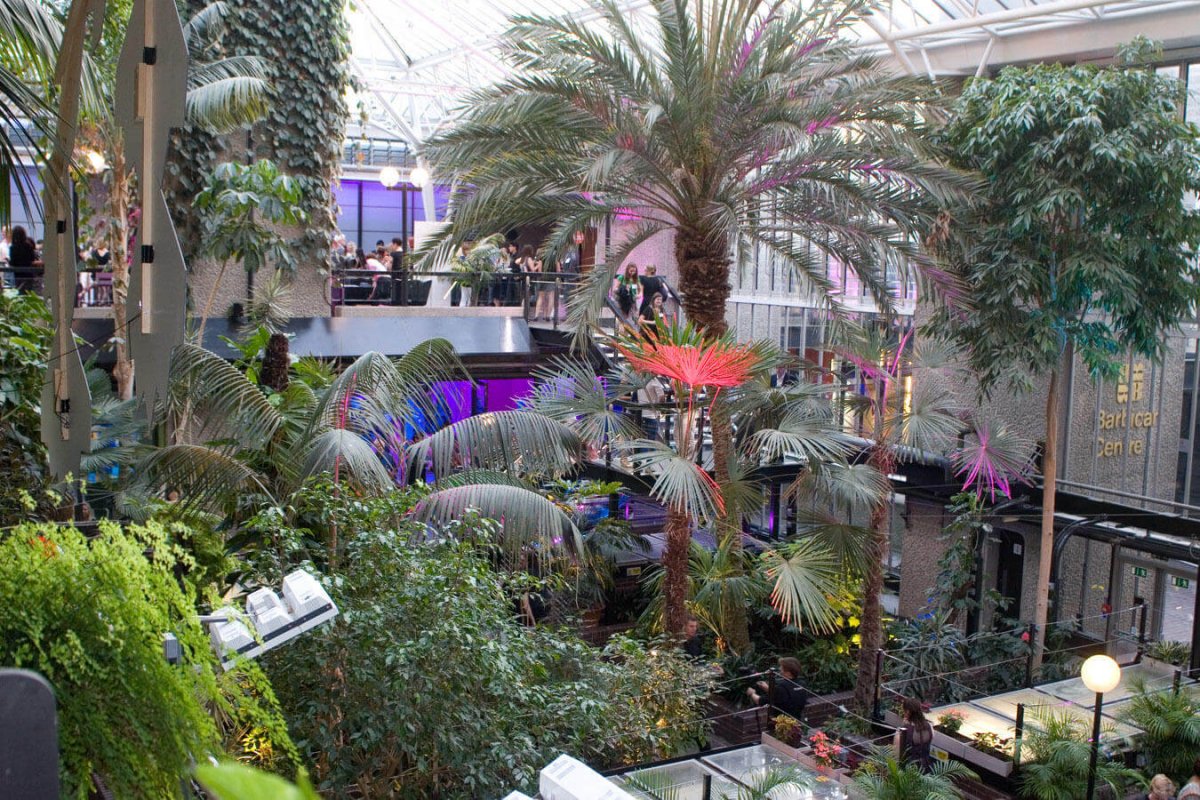The image depicts a large, multi-story indoor space resembling a conservatory or greenhouse, possibly within a conference or networking event. The area is filled with an abundance of tropical plants, including numerous palm trees, some of which appear to be illuminated with purple, pink, and red lights, creating a striking contrast among the predominantly green foliage. The structure features a predominantly glass roof, adding to the airy and open atmosphere of the setting.

From the vantage point of an upper floor, likely the second or third story, the camera overlooks both the lower levels and the vibrant greenery. People dressed in suits and dresses can be seen walking along the pathways that meander through the trees on the ground floor, while others congregate on what appears to be a balcony or second floor. A grand staircase connects the floors, allowing visitors to navigate the different levels.

Visible through a window on an upper floor is a wall displaying the text "Barbican Center" in gold metal letters, indicating the location. The glass walls and doors along the perimeter add to the sense of openness, blending the indoor space seamlessly with the outside world. The overall impression is one of a beautifully designed indoor garden, bustling with activity and enclosed within a modern, glass-ceilinged structure.